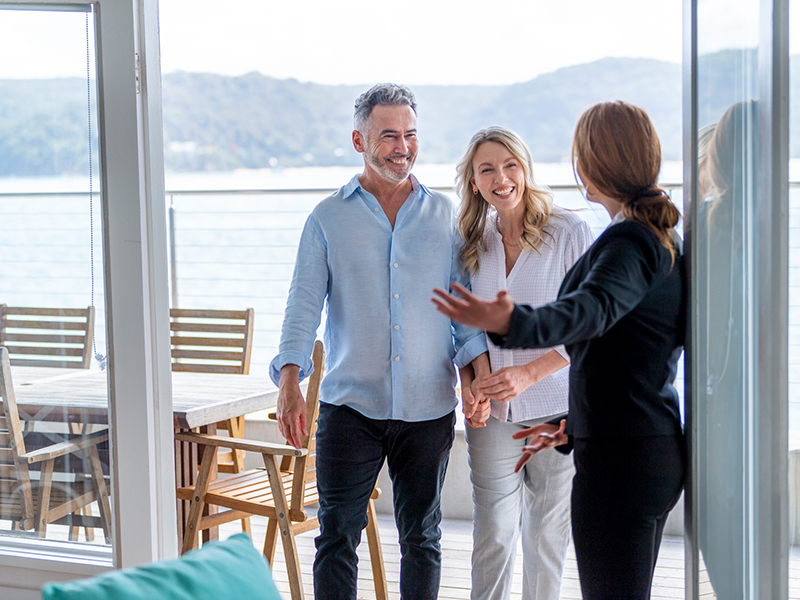The image is a color photograph capturing a middle-aged white couple being welcomed, possibly by a realtor, into what appears to be a waterfront building set against a scenic backdrop of hills or mountains. The couple is shown entering through an open framed glass door, which leads into an elegant interior. The man, distinguished with salt-and-pepper hair, a mustache, and a beard, is dressed in a blue Oxford button-down shirt and dark jeans, holding the hand of his partner. The woman, with long blonde hair, is wearing a white v-neck tunic-style shirt and khaki pants. Ahead of them, a woman with auburn hair pulled back in a loose bun, dressed in a formal black pantsuit, gestures with her left hand invitingly, emphasizing a welcoming atmosphere. Just outside the door, the deck features cable-style railing and is furnished with teak wood dining chairs around a matching table, enhancing the sophisticated lakeside or harborside ambiance.